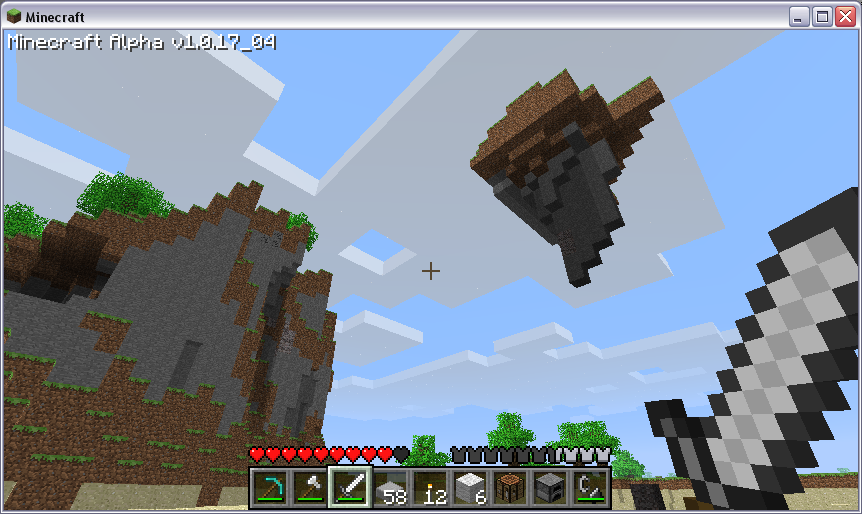This image resembles a scene constructed entirely out of tiny, interlocking plastic building bricks, evoking a pixelated, blocky aesthetic. In the forefront, there is a brightly colored panel at the bottom edge. Scattered above some of the symbols are vibrant red hearts, while the rest of the space features what appear to be rabbit heads. The captivating landscape showcases a variety of elements depicting trees, mountains, and rocks, rendered in a palette of greens, browns, greys, and whites, with blue representing the sky. The scene is rather surreal in its appearance. At the top, text reads "Minecraft Alpha," hinting at the early version of the popular sandbox game, Minecraft. An unusual object is noticed in the sky, adding to the enigmatic and intriguing nature of the image.